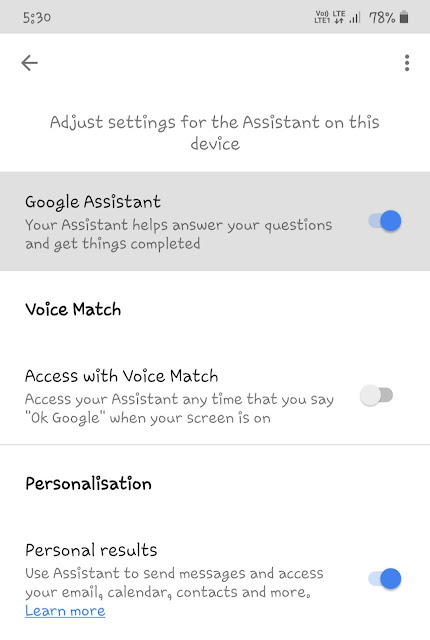The image depicts the settings interface for Google Assistant on a mobile phone. The screen shows the time as 5:30, with LTE signal bars and a battery life of 78%. The text on the screen features a playful, informal style with a somewhat squiggly, kiddish-looking font.

At the top, there is a title in gray, pencil-style text reading "Adjust settings for the Assistant on this device." The first highlighted option is "Google Assistant," with a description stating, "Your assistant helps answer your questions and gets things started." A blue toggle switch indicates that Google Assistant is activated.

Below this is the "Voice Match" option, described as "Access your Assistant anytime you say 'OK Google' when the screen is on." This feature is currently disabled, as indicated by the grayed-out toggle switch.

Further down is a section titled "Personalization" in black text. Within this section, the "Personal results" option states, "Use Assistant to send messages and access your email, calendar, contacts, and more." This feature includes a blue "Learn more" hyperlink and is turned on, as shown by the active blue toggle switch.

In summary, the image reveals that Google Assistant and personal results are enabled, whereas Voice Match is turned off.